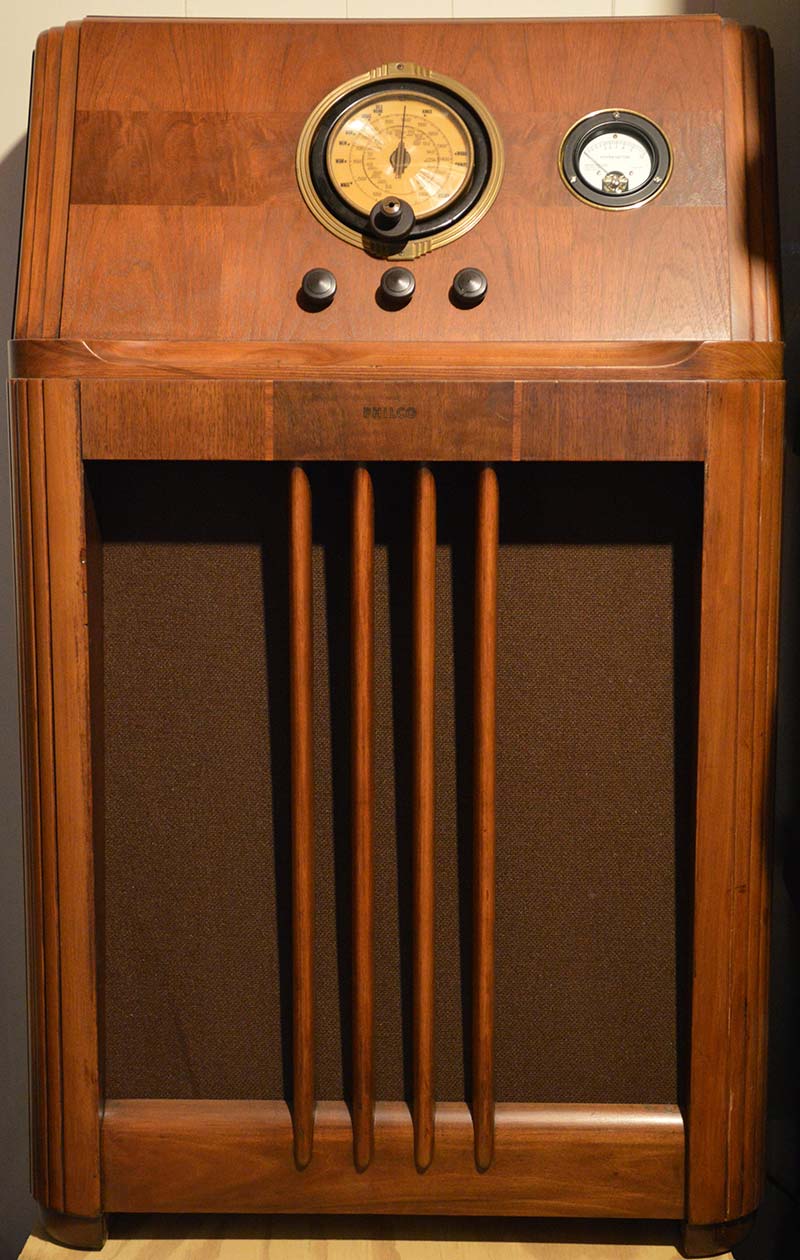This image depicts an old-fashioned, rectangular wooden radio, showcasing elements typical of the early models. The cabinet is crafted from fine, worn brown wood with intricate inlay work that presents varying textures yet maintains a smooth finish. The top third of the cabinet features a slightly forward-sloping section housing two prominent circular dials with glass covers. The dial on the left is larger and more intricate, featuring multiple rings of numbers and a full 360-degree readout. The right dial is smaller with a gauge-like display, resembling a 90-degree arc, possibly indicating different settings. Both dials are encircled by different trims—gold for the left and black for the right. Below these dials, a central knob is flanked by three smaller knobs lined horizontally. The lower portion of the cabinet recesses slightly to reveal the speaker area, marked by four vertical wooden bars. The overall finish of the radio, characterized by its worn brown color, adds to its vintage charm, making it a fascinating piece of historical electronic equipment.